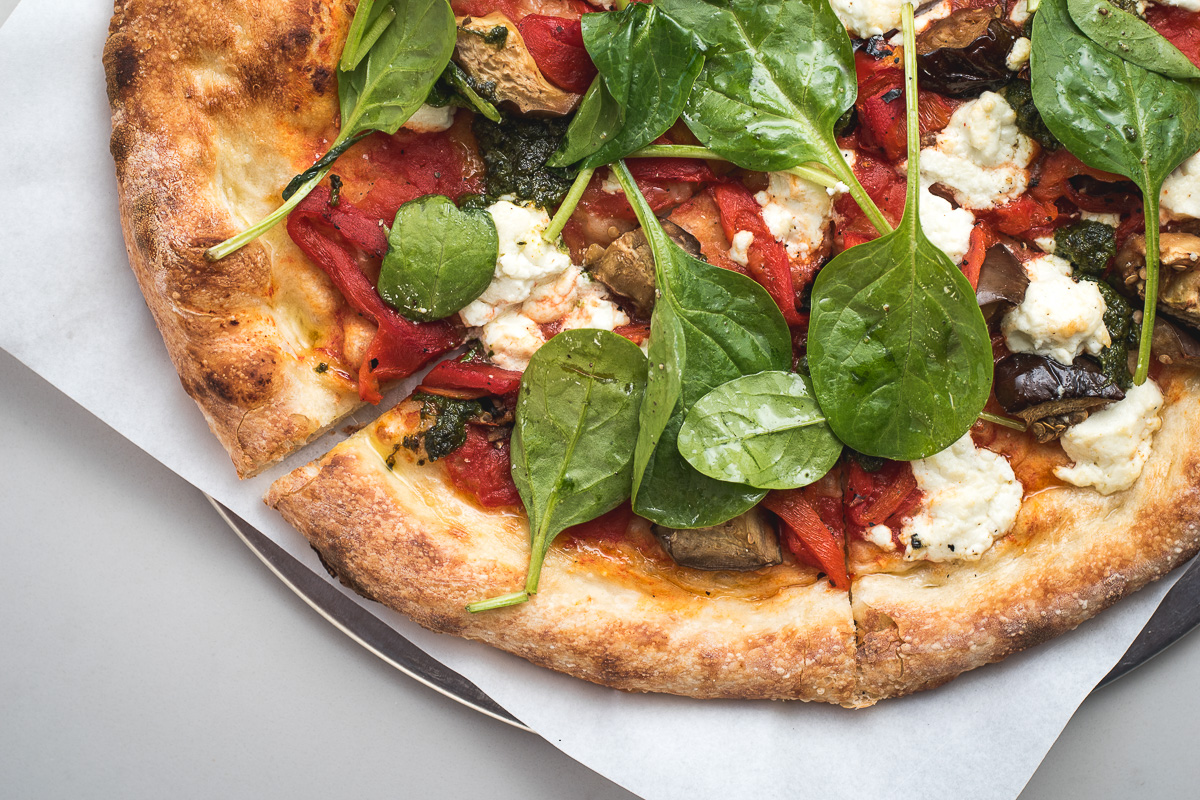This detailed, color photograph, taken in landscape orientation, captures a delectable, partially visible pizza, emphasizing its bottom half. Resting on a white piece of parchment paper on a round, silver-colored metal dish, the pizza is placed on a light gray tabletop. The pizza boasts a thick, golden-brown, bread-like crust with char marks around the edges. The exposed part reveals slices that have a cheese base smothered in tomato sauce, topped generously with mozzarella. It also features fresh vegetable toppings, including zucchini, uncooked baby spinach, and vibrant red peppers. Although some areas, particularly the top left portion, may appear sparse, the overall composition highlights the pizza’s inviting variety of colors and textures, presented through a style of photographic realism, typical of food photography.